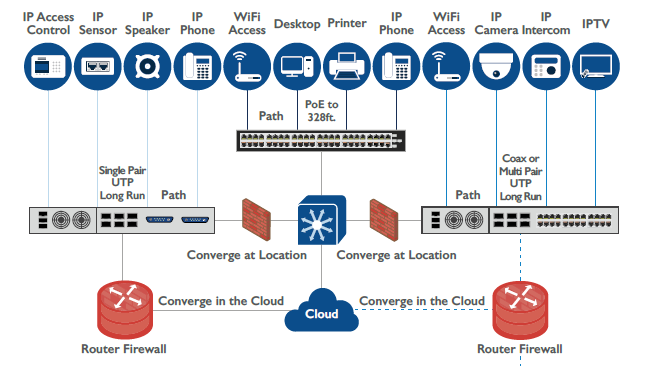The image is a detailed landscape diagram showcasing a cloud-based infrastructure with a focus on connectivity and data flow between various network components. Dominating the left and right sides are two representations of servers, detailed with visible serial and Ethernet ports, as well as fan grills. Hovering along the top, twelve blue circles each containing white icons represent various systems and devices such as IP Access Control, IP Sensor, IP Speaker, IP Phone, Wi-Fi Access, Desktop, Printer, IP Camera, IP Intercom, and IPTV. These icons are meticulously connected with blue lines to the two servers and a central PoE box, which also features Ethernet ports.

In the middle of the diagram, between the servers, the text highlights "Converge in the Cloud" and "Converge at Location," accompanied by cloud icons and further network symbols. The paths diverge into "Single Pair UTP Long Run and Path" on the left and "Coax or Multi-Pair UTP Long Run" on the right. The bottom section illustrates two router firewalls depicted as red cylinders with arrows extending outward, suggesting data directions. This intricate setup visualizes how various devices and control systems connect within a cloud-based network, delineating pathways for audio, visual, and control apparatus while maintaining a clear, albeit somewhat schematic, representation of modern computer network infrastructure.